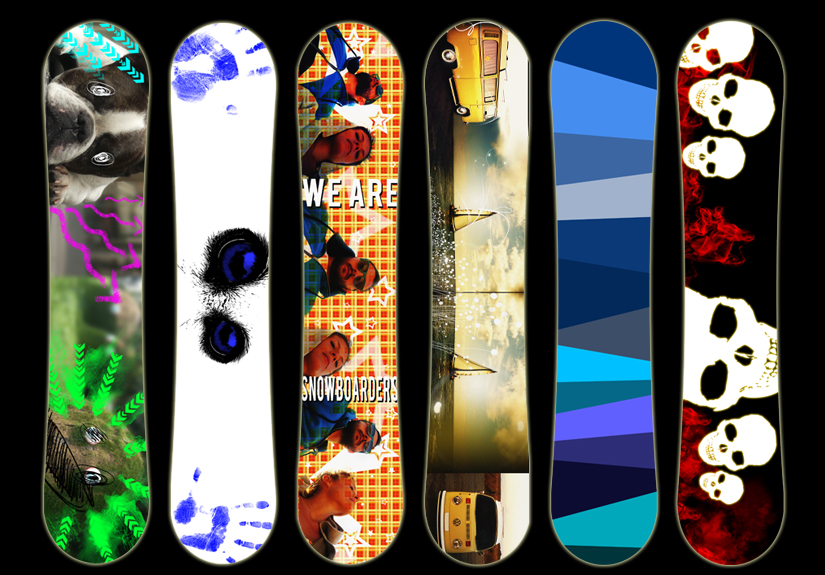This image showcases a lineup of six distinctive snowboards set against a solid black background. Arranged vertically from left to right, each snowboard displays a unique and eye-catching design:

1. **First Snowboard**: Features a vibrant and playful graphic with a Boston Terrier and an axolotl, surrounded by multicolored arrows of varying directions and sizes.
2. **Second Snowboard**: A white board adorned with a pair of eerie blue eyes, highlighted by a thick black outline, and accompanied by left and right handprints positioned at the top and bottom respectively.
3. **Third Snowboard**: Exhibits a red and yellow plaid pattern emblazoned with the phrase "We are snowboarders" in white. It also includes a series of people's faces arranged vertically along the board.
4. **Fourth Snowboard**: Depicts a serene scene featuring a Volkswagen bus parked near water, with two sailboats peacefully floating in the background.
5. **Fifth Snowboard**: A minimalist design composed of various shades of blue and gray, displaying sections of different widths.
6. **Sixth Snowboard**: A dramatic black background covered in flaming skulls, lending an intense and edgy flair to the board.